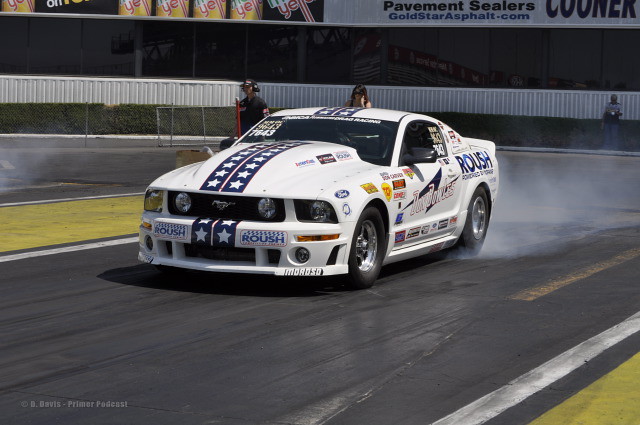This horizontally aligned rectangular image captures a dynamic race car, prominently displayed on a dark gray racetrack. The focal point is a striking white two-door Mustang adorned with distinctive blue stripes running along its elevated hood and roof. Each stripe is filled with white stars, creating a patriotic and eye-catching design. The front bumper features the word "Roush" in bold letters, while the back also displays "Roush" in large blue letters. 

The car, seemingly in motion with exhaust fumes visible behind it, is decorated with various logos and advertisements in blue, yellow, and reddish hues along its sides. Though many of the side writings are too small to read, the detailed sponsor logos include 'Yelp', 'Pavement Sealers', and 'Goldstarasphalt.com'. In the background, a white and gray building stands with banners, adding to the race track ambiance. A man in a black shirt, hat, and headphones stands attentively by the sidelines, along with a woman watching the spectacle. Fine print in the lower left corner reads "D. Davis Primer Podcast", adding a layer of detail to the overall scene.